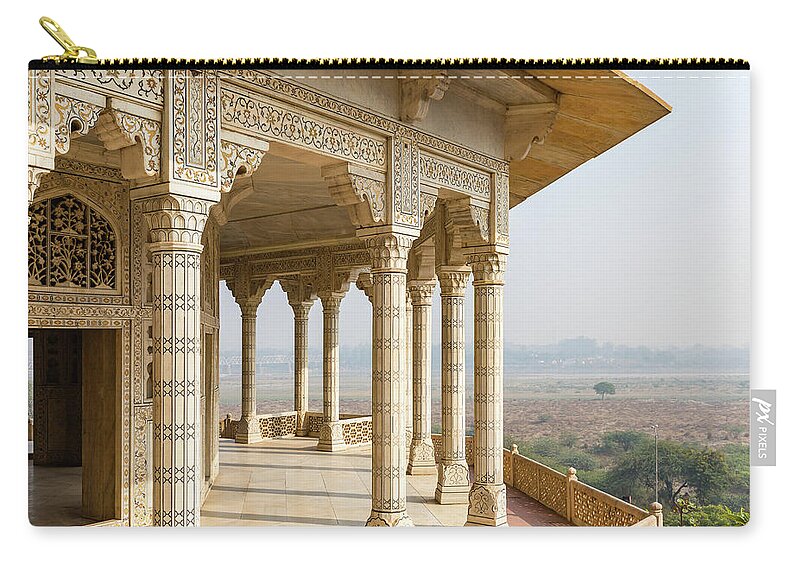This image depicts a detailed handbag or coin purse adorned with an outdoor landscape. The primary focus of the design is an ornate Middle Eastern or Islamic building, featuring gold and dark brown inscriptions, intricate detailing, and numerous columns. The building spans from the top left to the center of the image, set against a backdrop that includes a skyline, mountains, and green fields to the right. The sky is gray, fading into the distance. The pouch has a zippered top with a gold zipper pull and a small gray tag on the bottom right that reads "PX PIXELS" in white print. Additionally, there is a green tree visible in the bottom right corner, adding to the picturesque scene.